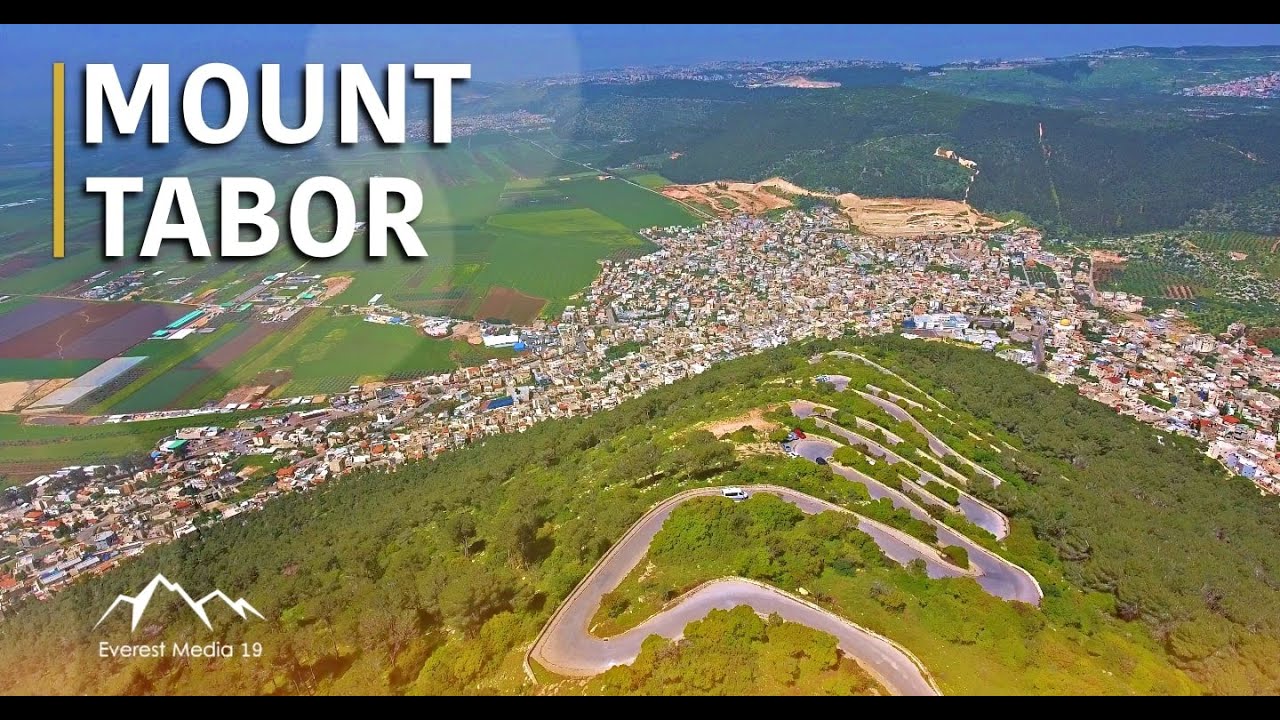The aerial image prominently features Mount Tabor, identified in bold white text on the top left, with "Everest Media 19" and a mountain logo at the bottom left corner. The centerpiece is a serpentine road that crisscrosses the green, tree-covered ridge in multiple S-shaped curves, snaking down the mountainside. As the road descends, it leads into a densely packed urban area where the houses are so closely clustered that it seems one could reach out a window and hand a cup of milk to a neighbor. Beyond this urban sprawl, the landscape shifts sharply into farm fields and eventually to a mountain range stretching into the distance under a blue sky. The intricate layout of the road, flanked by rich foliage, contrasts strikingly with the dense, maze-like arrangement of buildings, creating a vivid and detailed depiction of the diverse terrain.